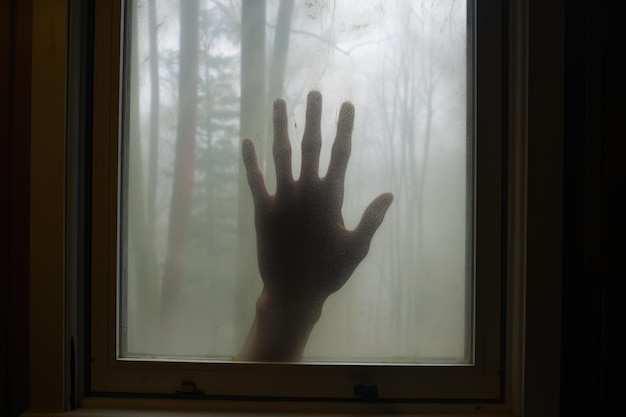The image depicts a haunting scene that appears to be a still frame from a horror movie, captured in a color photograph. Taken from inside a house, the photo focuses on a window with a white frame and lath work around its edges. Pressed against the window is the smudged palm of a man’s hand, fingers spread wide, giving the chilling impression that he is desperately trying to get in. The glass is slightly fogged, adding to the eerie atmosphere. Outside the window, the background is muted and ominous, featuring a blend of neutral colors—black, white, gray, and brown—interspersed with some green. Tree trunks and a mix of pine trees and leafless trees are visible through a heavy mist, making the scene appear desolate and foreboding. The overall effect is intensely creepy, perfectly capturing the unsettling essence typical of horror themes.